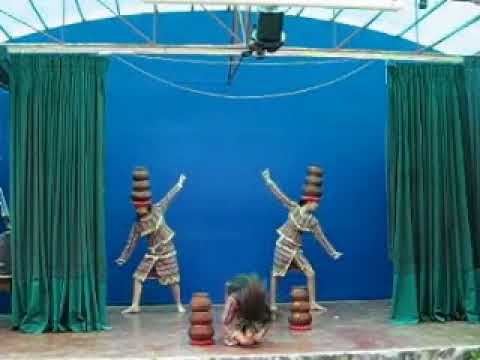In this detailed photograph of a stage setting, the backdrop is a vibrant blue with heavy green curtains hanging from the ceiling structure on both the left and right sides. Center stage are two performers, positioned side by side, each wearing matching patterned outfits consisting of long-sleeved shirts and skirts. They are adorned with unique, tall hats that resemble three pots stacked on top of each other. Their poses are distinctly theatrical: each performer extends one arm out to the side while bending their knees, leaning in opposite directions as if caught mid-motion.

Between these two main characters, there is an additional performer kneeling on the floor, bent over with their face towards the ground, suggesting a dynamic scene. This person is aligned with the others, also dressed in a matching outfit and hat. Scattered in front of the performers are similar hat-like objects, placed on the brown and gray mottled floor of the stage. Additionally, there are structures resembling green grass growing out of the floor, adding to the whimsical nature of the set. Above, a curved metal framework supports a lighting rig, illuminating the entire scene with a theatrical glow.